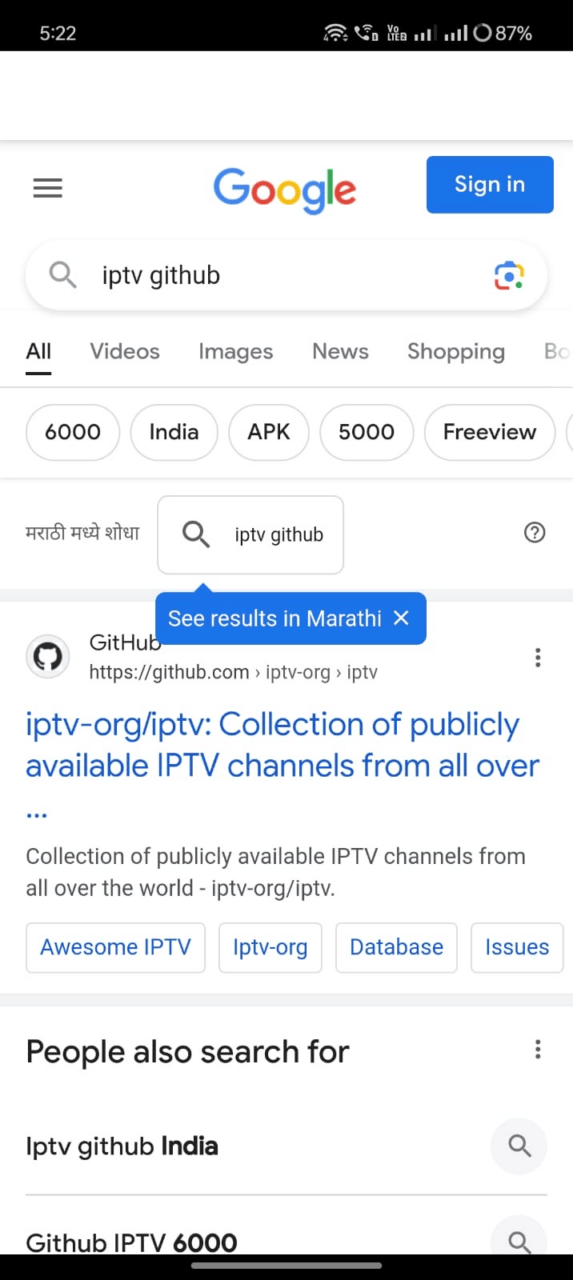The image depicts a Google search results page accessed on a mobile device, as evidenced by the visible indicators at the top of the screen, which include the time displayed as 5:22, Wi-Fi signal strength, and battery percentage. The screenshot captures a Google search for "IPTV Github," with the user navigating the search engine on their phone. A blue "Sign in" button is prominently featured at the top-right corner, offering the option to access a personalized Google account.

Below, the search results interface displays the typical tabs: All, Videos, Images, News, and Shopping, with the "All" tab currently highlighted. The results count indicates approximately 6,000 hits related to the query. Some targeted content mentions India and APK files, suggesting an interest in specific regional or application-based information. An option to see results in Marathi, a regional Indian language, appears on the left, accompanied by script characters indicative of the language.

The first search result is a link to Github, described as a "Collection of publicly available IPTV channels from all over the world." This description hints at a repository of Internet Protocol Television (IPTV) resources that are accessible to the public. The image likely aims to highlight the process and content of the search, focusing on how users can find IPTV resources on Github.